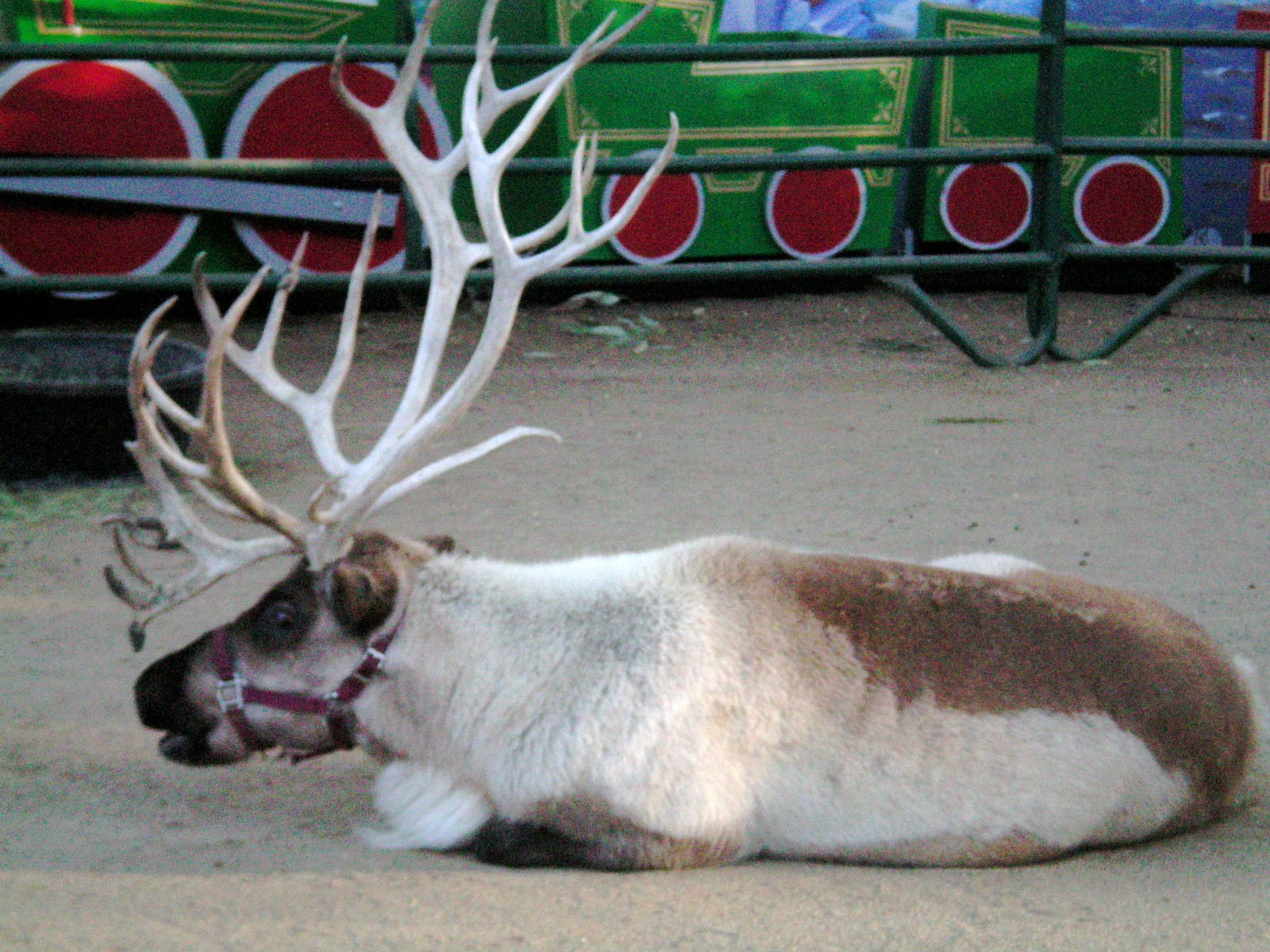In the center of this rectangular photograph, taken in natural daylight at what appears to be a fair or petting zoo, a mostly white reindeer with brown spots is sitting on a sandy, rocky ground. The reindeer, which has large, multi-pointed antlers and a red halter around its head, casts a shadow, indicating the sunlight is coming from the top right. Adjacent to the reindeer is a large black feed or water bowl, surrounded by some green hay. Just beyond the reindeer, a green metal gate, typical of an outdoor petting zoo pen, secures the area. In the background, a small carnival-like train with red wheels and green, variably-shaped cars is visible. The photograph captures a vivid scene with colors including tan, black, brown, white, red, green, and blue, emphasizing the outdoor setting and the charm of the zoo environment.